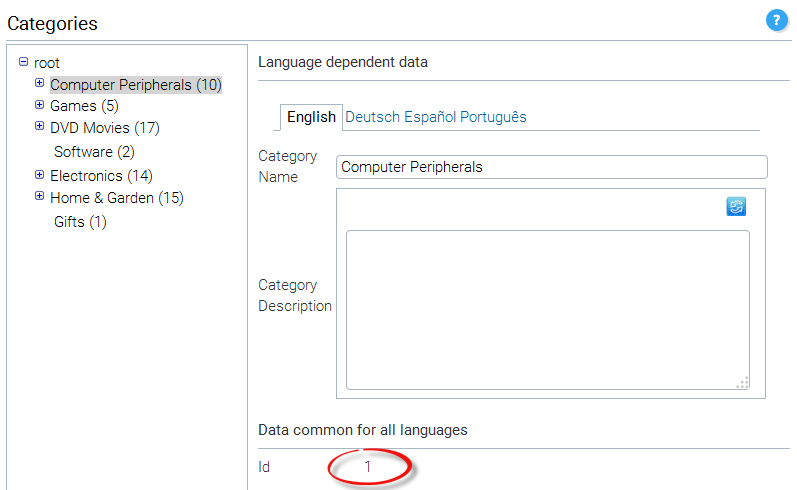This image is a screenshot of a digital interface, which could be either an application or a website, though it is unclear from the image alone. The interface is characterized by its minimalist design, featuring a white background and simple gray lines that delineate different sections.

On the left side of the screen, there is a hierarchical tree menu displaying various categories. The root category is expanded and reveals five subcategories: Computer Peripherals, Games, DVD Movies, Software Electronics, Home and Garden, and Gifts. Each of these subcategories has a plus button next to it, allowing further expansion into more specific subcategories.

To the right of the tree menu, there is a section titled "Language-Dependent Data." Here, users can choose the display language from options including English, Deutsch, Español, and Português, with English currently selected. Beneath this language selection, there is an input field labeled "Enter Category Name," which is currently focused on the "Computer Peripherals" category. There is also an option to add a category description within this section.